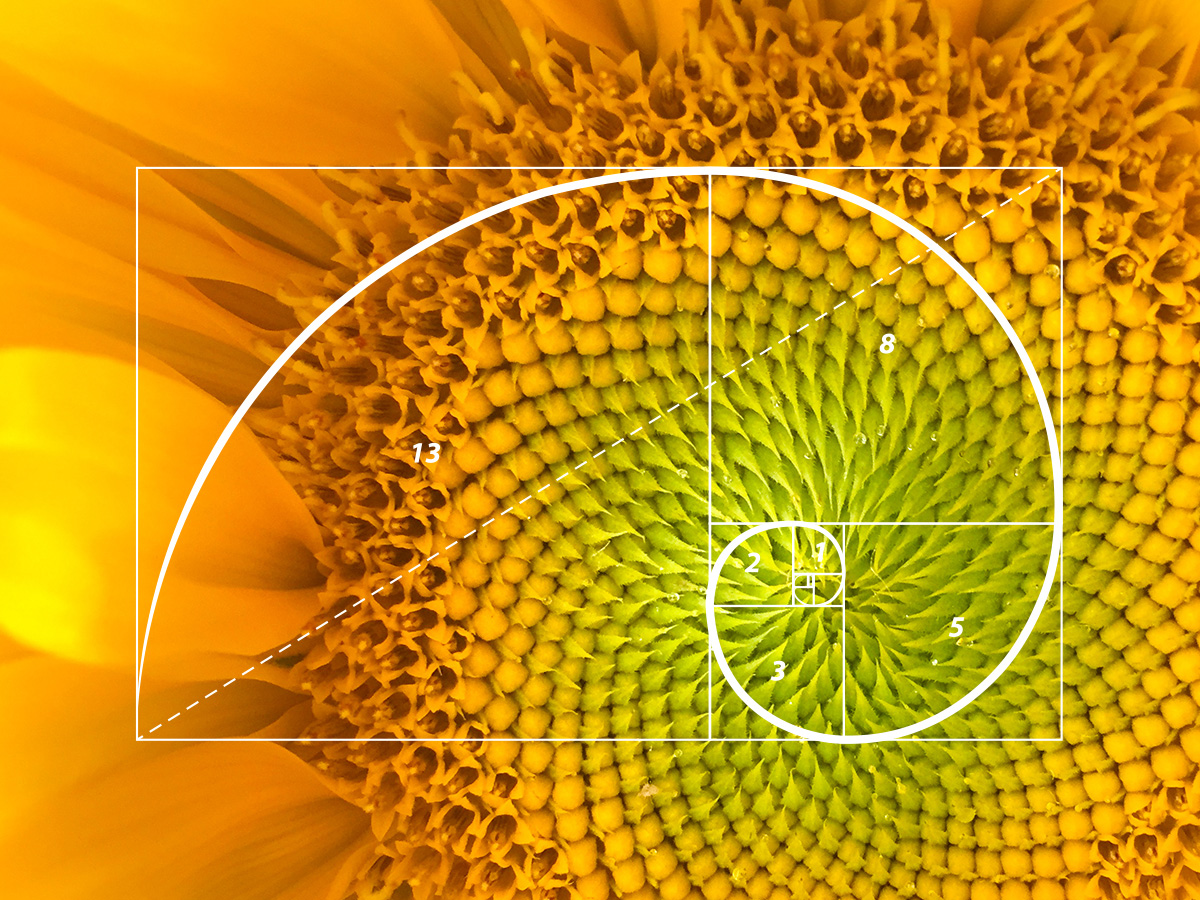The image is a detailed, close-up of the inside of a flower, possibly a sunflower or daisy, showcasing a vibrant array of yellow and orange petals surrounding a multitude of small, intricate seeds. The flower's center features a combination of yellow bulbs transitioning into green ones. Superimposed on this organic background is a geometric design consisting of a rectangle with a bold curve that intertwines through it like a wave, accompanied by a dotted line running diagonally from bottom to top. This rectangle is divided vertically, with the left side marked with the number 13 and the right side with the number 8. Below the 8, there is an additional square containing the numbers 5, 3, and 2. The geometric overlay adds an intriguing contrast to the natural intricacies of the flower, with the dotted line and numerical annotations further enriching the visual complexity of the image.